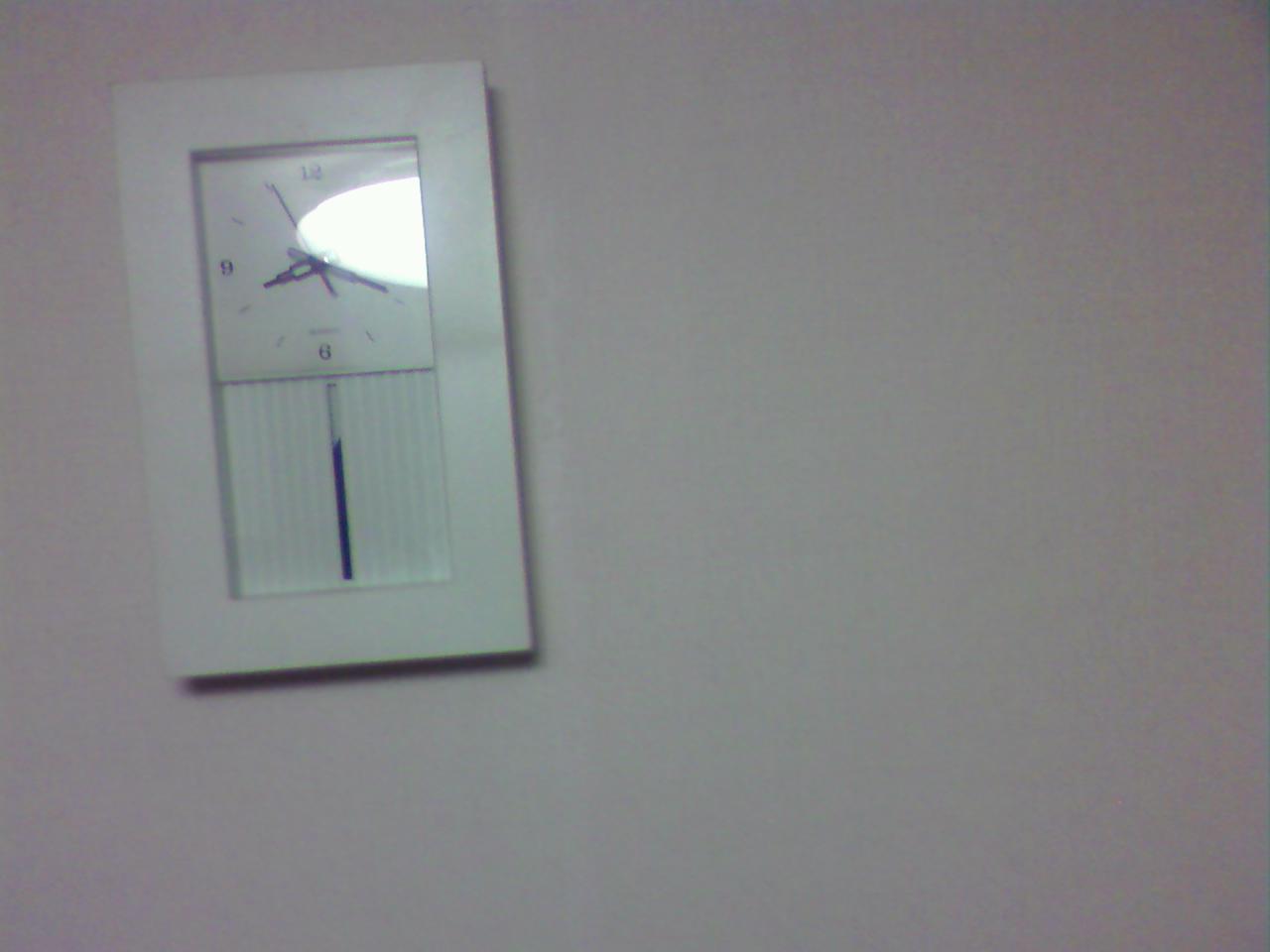This low-quality snapshot photograph captures the image of a white wall occupying the majority of the frame. The entire right half of the image is completely white, offering no discernible details. To the left side of the image, partially towards the center, there is a vertically-rectangular clock with a white border. The clock is slightly tilted to the left.

The clock face is modern with a reflective square glass cover, through which the reflection of an overhead ceiling lamp or light is prominently visible, creating a bright glare. The clock's design features two square sections stacked vertically, framed by a white border. The upper section houses the clock face where the numbers 12, 9, and 6 are clearly visible, while the hour, minute, and second hands point to approximately 8:20. Directly below the clock face, the lower square section appears corrugated, resembling a stage curtain. The overall presentation of the elements within the image lacks sharp details due to the low-quality nature of the photograph.